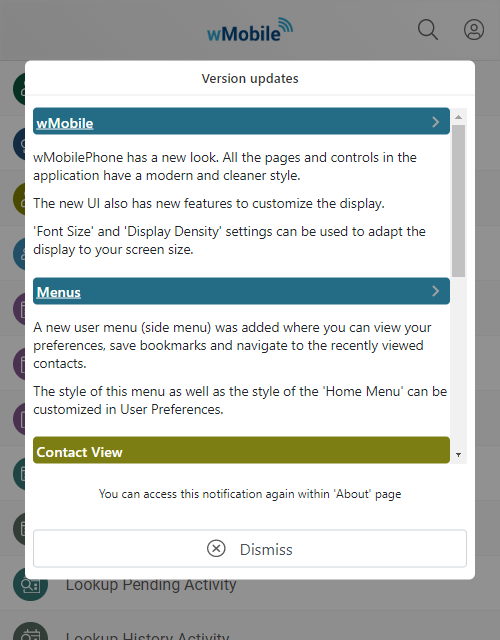This image is a vertical, rectangular screenshot of a version update notification for the W-Mobile application. The background is gray and blurred, with the word "W-Mobile" visible behind a large white rectangular overlay. The notification announces that W-Mobile has a new, modern, and cleaner look. All pages and controls within the application have received a style update, and new UI features allow users to customize their display settings, including font size and display density, to better fit various screen sizes. 

A new side user menu has been introduced, allowing users to view preferences, save bookmarks, and navigate recent contacts. Both the new side menu and the home menu styles can be customized in user preferences. The notification mentions that this message can be accessed again from the about page. At the bottom of the notification, there's a dismiss button represented by a circle with an "X" in it.